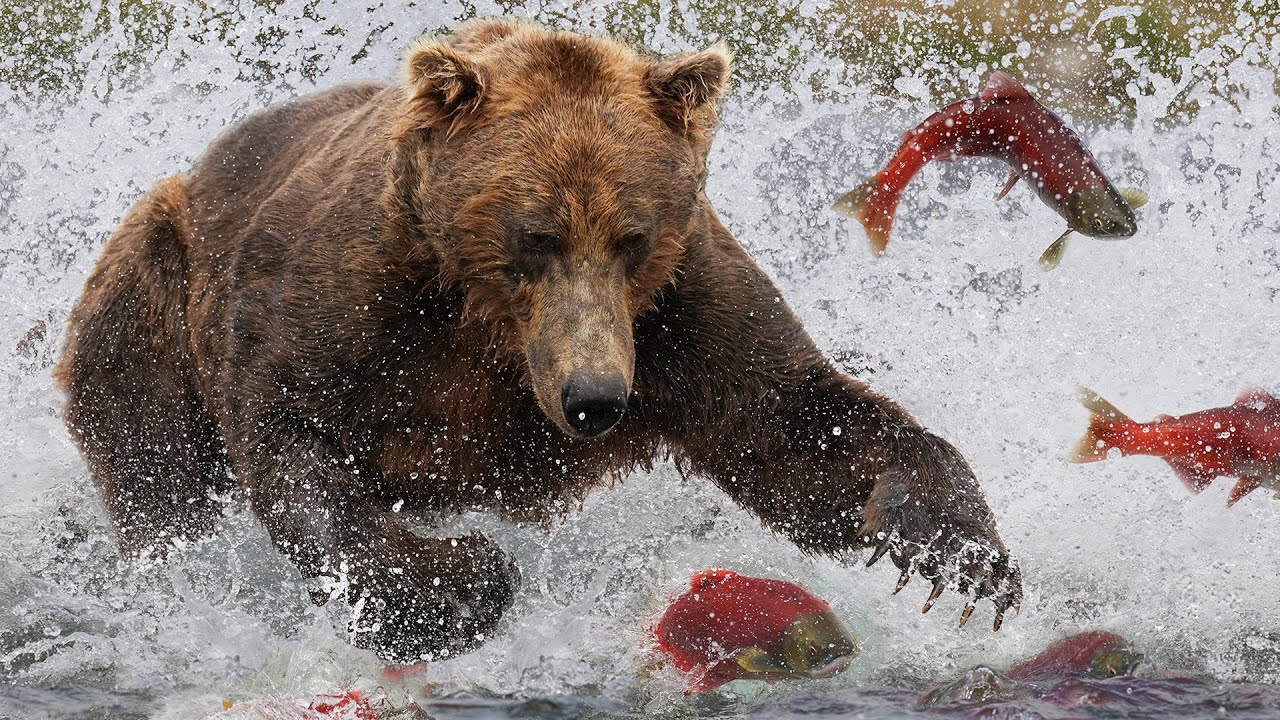In this dynamic nature photograph, a determined brown bear charges through the water, creating a massive splash that cascades across the entire image. With its paw outstretched and claws bared, the bear's focus is intensely locked on a vibrant, bright red salmon directly below its paw. The salmon, distinguished by their vivid red bodies and green-tinted faces and fins, are in a frantic scramble to escape. One salmon, captured mid-leap with an athletic half-body curl, arcs gracefully over the bear's shoulder, seemingly eye-level with the predator in a desperate bid for freedom. Another fish is a foot above the water, streaking horizontally away, while additional salmon dart beneath the surface, adding to the chaotic scene. Surrounding the action are splashes and bubbles, testament to the bear's powerful plunge and the ensuing frenzied escape of the salmon. Hints of green in the blurred background suggest a lush, natural setting, though obscured by the sheer energy and movement of the moment.